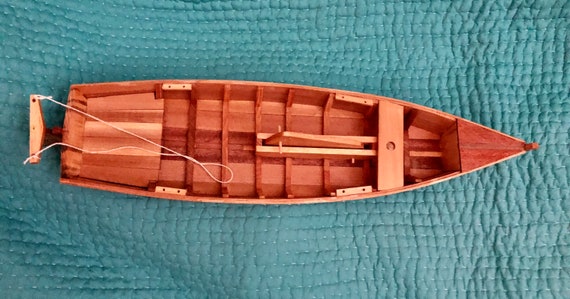This top-down photograph captures a highly detailed, handcrafted wooden rowboat model, resting on a turquoise blue quilt. The boat, appearing in a reddish-brown, rust color, is intricately constructed with ribbing on the inside, showcasing meticulous craftsmanship that would require great precision and care to assemble. The slender boat shows panels running both horizontally and vertically, suggesting fine detail work and adding to its realistic appearance. 

At the back of the boat, a thin white thread is attached where a rudder or motor would typically be, indicating a mechanism to control the direction of the boat. The absence of oars or any visible propulsion system further emphasizes its model nature. The boat's design includes a pointed bow and a straight stern, with seating for two, highlighting the small scale that might easily be mistaken for a toy. No other objects or texts are present in the image, ensuring the viewer's focus remains entirely on the expertly crafted wooden rowboat and its quilted backdrop.